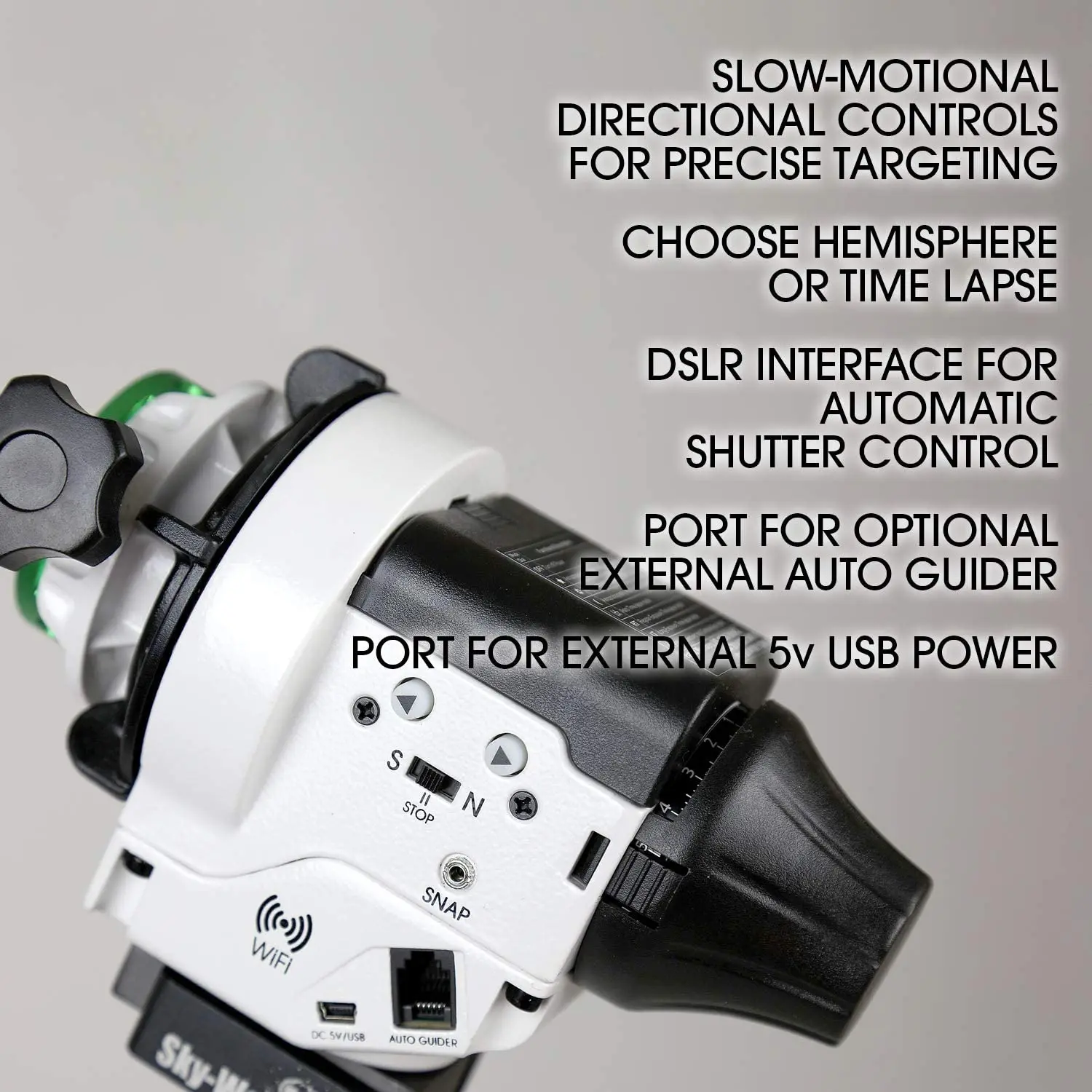The image depicts a sophisticated camera-like device, possibly a camera microscope or a specialized imaging tool, featuring a sleek design with a white and black exterior. The device prominently includes a black lens surrounded by black plastic, and it has various control buttons and ports. On one side, there are directional controls including forward and backward buttons, left and right arrows, as well as an S (presumably for South) and N (for North) button, beside a switch labeled "Stop" in the middle. Additionally, there is a Wi-Fi indicator, suggesting wireless connectivity.

The side of the device has multiple ports, including one labeled "DSLR Interface for Automatic Shutter Control," a port for an "Optional External Auto Guider," and another for "External 5V USB Power." Plug-ins for micro-USBs and internet cables are visible, indicating its ability to interface with various external devices and accessories. The device also features labeled text in black, stating: "Slow Motion Directional Controls for Precise Targeting. Choose Hemisphere or Time Lapse."

The background of the image is a plain white, emphasizing the device as the focal point, while the detailed black text overlay adds informative context about the device’s advanced features and connectivity options.